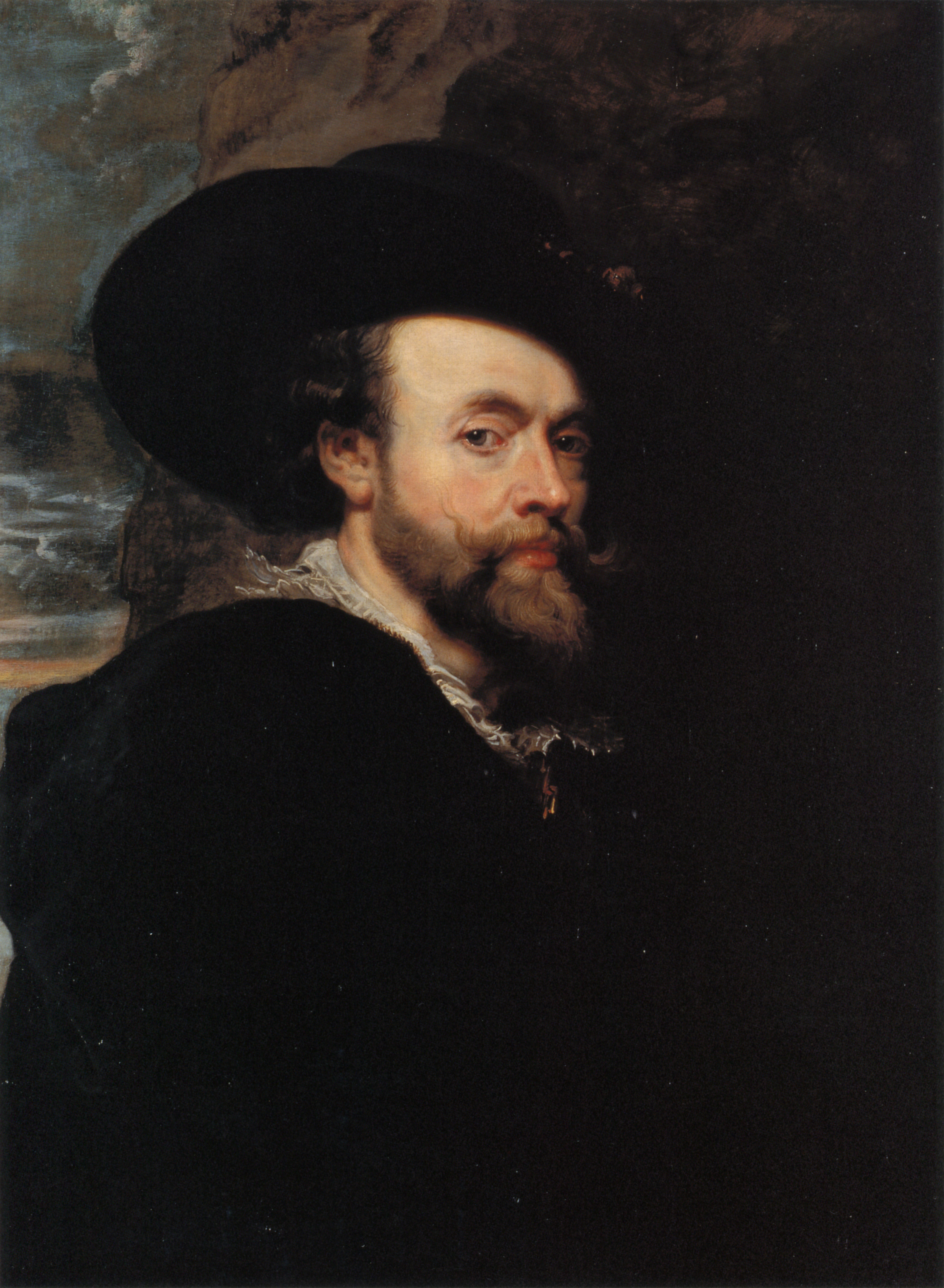This detailed portrait painting, likely from the 14th to 16th century, features a middle-aged white man gazing directly at the viewer with an inquisitive, yet somewhat apprehensive expression. He sports a distinctive mustache that curls up at the ends and a long, brown beard extending from his chin. His attire consists of a wide round black cap and a long black robe or cloak, potentially similar to a priest's garment, with a glimpse of white clothing — possibly a scarf or shirt — underneath. The background is almost entirely black, so his dark clothing blends into his surroundings, though there is a hint of dark brown and multicolored textures suggesting a worn or damp environment. His bright red lips stand out vividly against his solemn attire.